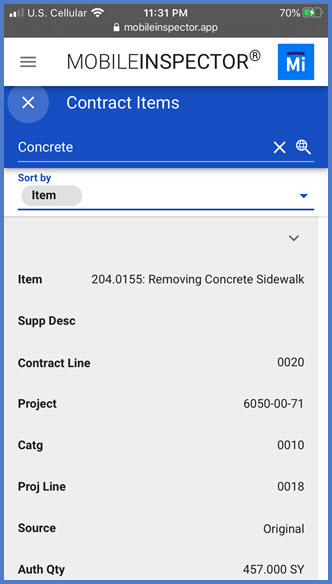The image captures a screenshot of the MobileInspector app. At the top of the app interface, the domain "mobileinspector.app" is prominently displayed. Directly below, a white header features the app's name, "MobileInspector," accompanied by a blue square logo with the initials "MI" in it. 

Underneath the header is a blue section titled "Contract Items," within which the word "concrete" is listed. This section is followed by an option labeled "Sort By" with a drop-down list intended for item selection.

The lower segment of the screen transitions to a light gray background, detailing specific contract information. The item specified is "204.0155: Removing Concrete Sidewalk." Below this, an option labeled "SUPDSC" is visible, though its function is unclear. Additional contract details include:
- Contract Line: 0020
- Project: 6050-00-71
- CATG: 0010
- Project Line: 0018
- Source: Original
- Authorized Quantity: 457.000 SY